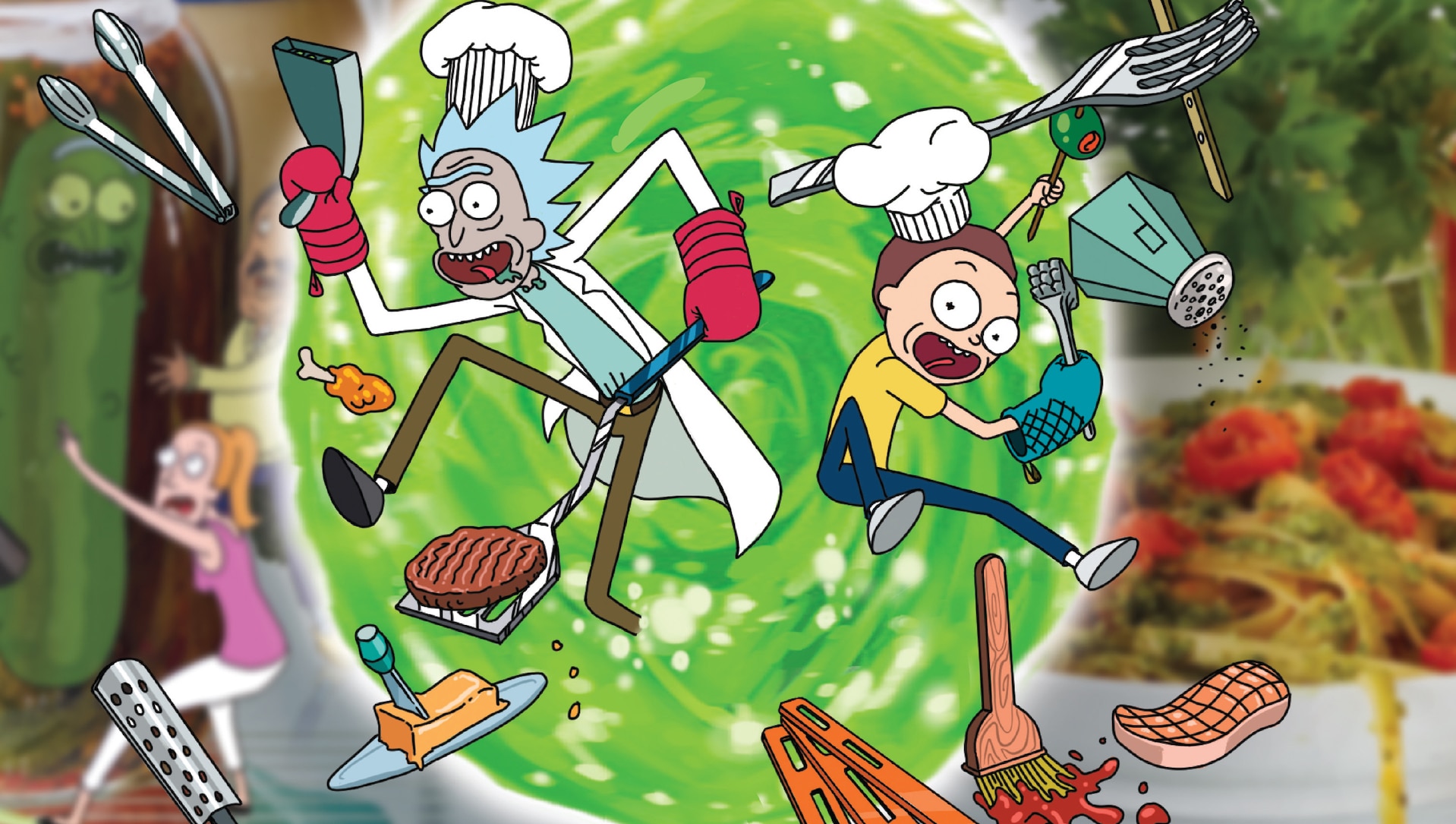This illustrated image features the characters Rick and Morty from the TV show "Rick and Morty" in a whimsical culinary setting. On the left is Rick, an older man with spiky gray (or blue) hair, wearing a white lab coat, light teal shirt, brown pants, black shoes, a white chef's hat, and red oven mitts. He holds a spatula with a burger on it in one hand, while the other wields a peculiar gun-like device. To the right stands Morty, a younger boy with short brown hair, in a yellow shirt, blue jeans, white shoes, and a blue oven mitt. Morty also sports a chef's hat and holds a meat tenderizer in one hand and an oversized toothpick with a giant olive in the other. 

They appear to be emerging from a large, green, swirling portal in the background, accompanied by various airborne kitchen utensils and food items like a giant fork directly above Morty, a cucumber with facial features on the left, and a myriad of other detailed kitchen-related imagery. Some additional elements include a blurry figure of a scared woman with yellow hair and a pink shirt, a meat grater, a fork above Morty, a salt shaker, a picture of a steak, a pastry brush, and what looks like some salad with tomatoes and pasta on the right side of the image. The overall scene is chaotic yet vividly animated, capturing the essence of a culinary adventure bursting out of a cosmic rift.